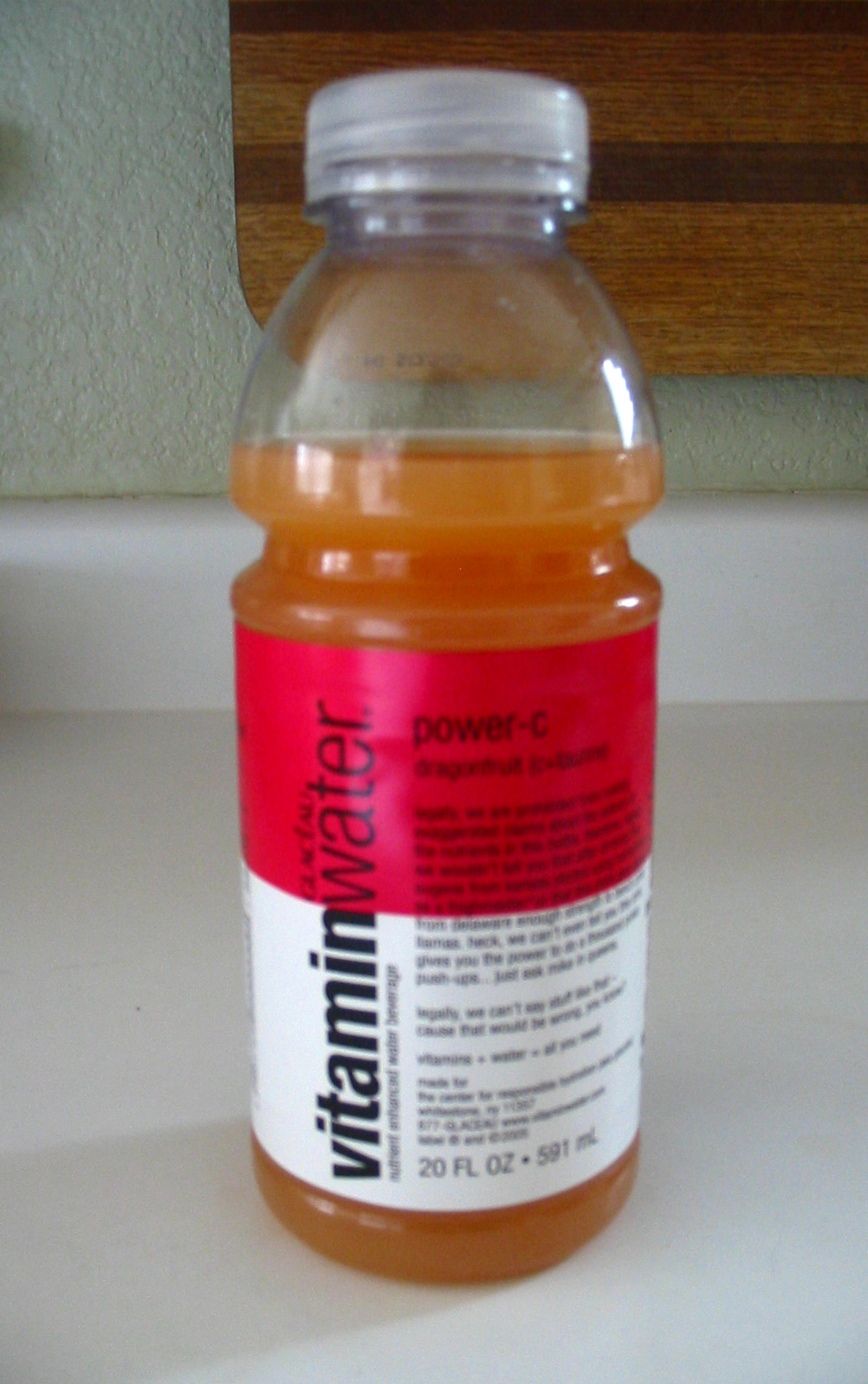In this soft color photograph, a clear plastic bottle of Vitamin Water stands upright on a white countertop, partially filled with a peach-colored liquid that evokes a light orange hue. The bottle is topped with a semi-transparent white lid, securely screwed on. The label on the bottle is divided into two sections: the top half is red, while the bottom half is white. Written vertically on the left side of the label are the words "Vitamin Water" in black text, and horizontally nearby is the bolded text "Power C" followed by "dragon fruit." Additional information and ingredients are listed in small black font beneath this primary text. In the background, the white countertop is bordered by white trim, and behind it is a white concrete wall with a cut-out section revealing a wooden grain frame, potentially part of a decorative or structural element. The measurement of the liquid is clearly marked on the label as "20 fluid ounces (591 milliliters)."